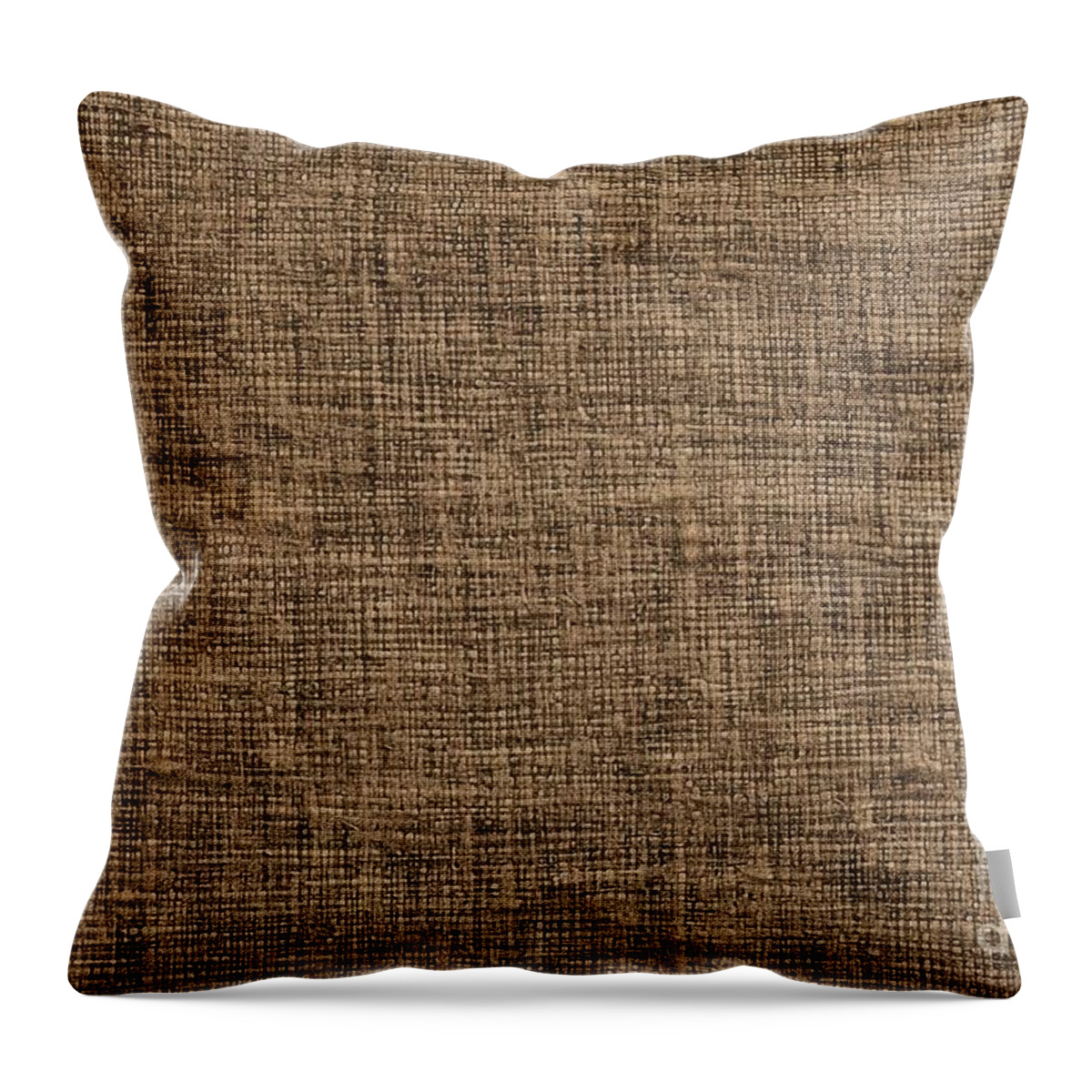This is a detailed color photograph of a textured, square pillow with a rustic burlap or linen-like appearance, photographed against a plain white background. The pillow fabric is a mix of light brown, medium brown, and dark brown fibers, creating a variegated, non-uniform look. The woven fibers run vertically and horizontally, reminiscent of a potato sack design, giving it a rough and textured appearance. The corners of the pillow are pointy, and the edges curve inward slightly, causing the pillow to slouch a bit as if it were bending at the waist. Along the right vertical edge near the lower corner, a small gray or white tag protrudes from the side, but no text is visible on it. Additionally, just above the tag, there is a small white circle. The pillow casts a shadow beneath it on the white surface, enhancing the simplicity of the background. This visually interesting pillow would be suitable as a decorative piece on a couch rather than for sleeping.